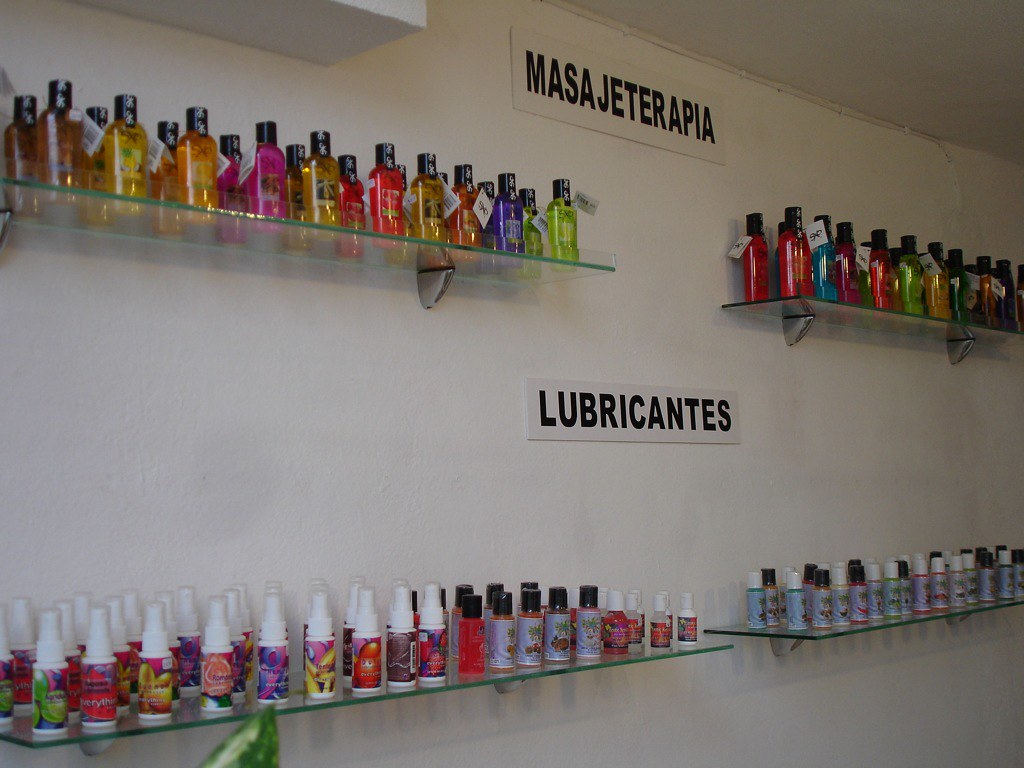The photograph captures a white wall adorned with four glass shelves, each holding an array of bottles containing liquid products. Some bottles are designed as spray containers, while others come with screw caps. The bottles are of various vivid colors, including bright green, bright red, bright yellow, and magenta. Centrally placed between the two sets of shelves are two signs in a dark black font, written in another language: "Massageterapia" and "Lubricantes," indicating that the lower shelves contain lubricants. The setting appears to be a store. At the bottom of the image, a decorative plant leaf is visible next to one of the shelves, adding a touch of greenery to the scene.